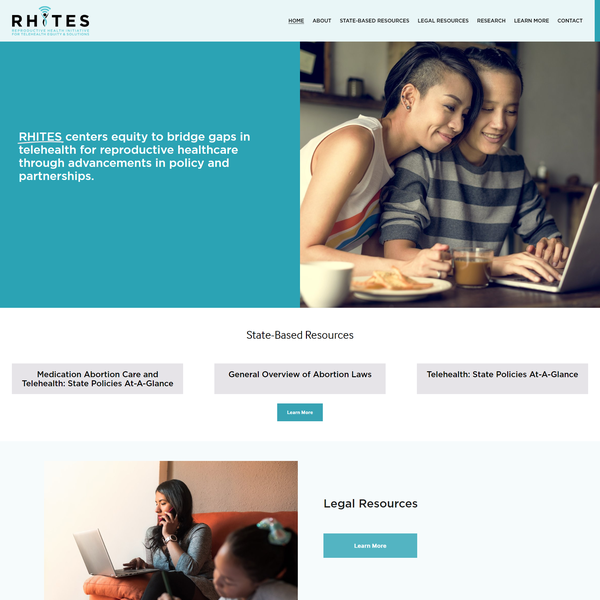The image features a detailed layout with the following elements:

1. In the left top corner, the text "R-H-I-T-E-S" appears in black.
2. The top of the page is adorned with a light blue band stretching across the entire width.
3. Starting from the middle and extending to the right within the blue band, navigation links in black font read: "Home," "About," "State-Based Resources," "Legal Resources," "Research," "Learn More," and "Contact."
4. On the left side of the image, there's a teal square with white font, presenting the text: "Rights Center, Equality to Bridge Gaps in Telehealth for Reproductive Health Care through Advancement in Policy and Partnerships."
5. On the right side, an image depicts a child and an adult (possibly a mother or sister) both with dark hair, looking at a laptop. The child wears a gray striped t-shirt, and the adult is in a sleeveless t-shirt.
6. Below the main imagery:
   - "State-Based Resources" is highlighted.
   - A gray button with black font is labeled "Medication, Abortion Care, and Telehealth State Policies at a Glance."
7. To the right of this:
   - A button labeled "General Overview of Abortion Laws."
   - Another button labeled "Telehealth State Policies at a Glance."
   - Each button is distinguished by theme and placement.
8. Centered below these buttons is a teal button labeled "Learn More."
9. Midway down the page, "Legal Resources" is displayed.
10. Beneath this, another teal "Learn More" button is positioned.
11. To the left of the "Legal Resources" section, there is another photograph featuring a woman working on a laptop with a small girl.

This intricate layout highlights the importance of providing accessible information on reproductive health care through telehealth advancements, supported by an array of visually organized resources and links.